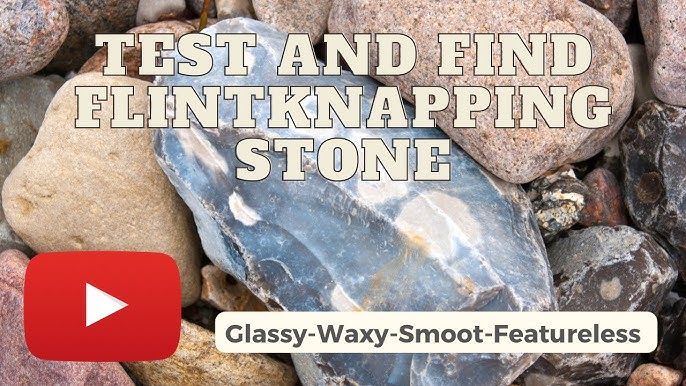**Descriptive Caption:**

The thumbnail for a YouTube video prominently features the platform's recognizable red box with a white, right-pointing triangle indicating the video play button. Superimposed on the image in a beige-colored font is the instructional text: "Test and Find Flint Knapping Stone," with the phrase "Flint Knapping" distinctly spelled out as F-I-L-N-T-K-N-A-P-P-I-N-G. At the bottom of the thumbnail, a light-colored text box contains dark lettering that reads "glassy/waxy smooth, featureless," though the word 'smooth' appears to have a typographical error, being written as "S-M-O-O-T." The background is comprised of a pile of diverse unpolished raw stones, displaying shades of gray, beige, red, and almost black, providing a rugged and authentic context to the instructional content.